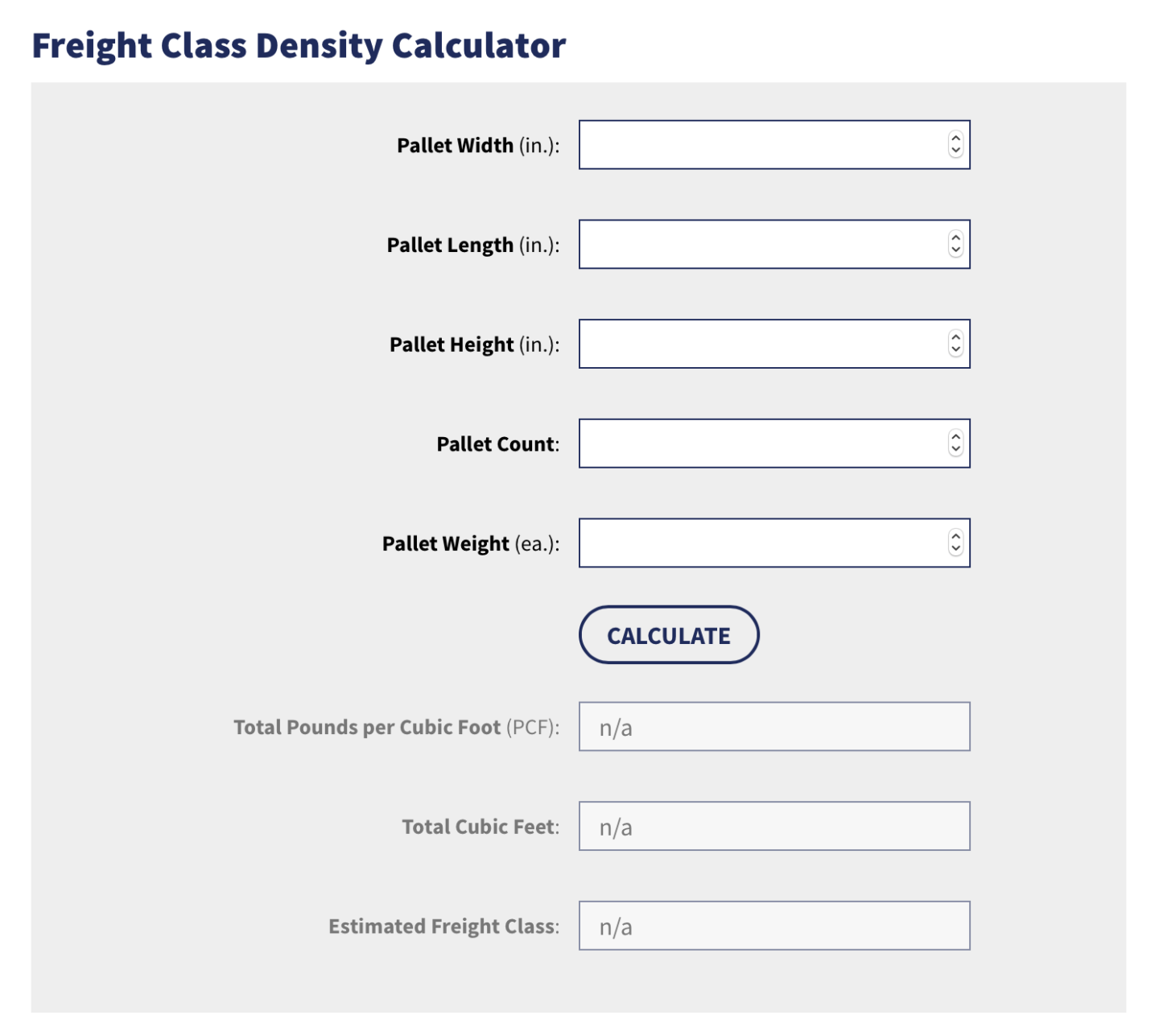The image displays a freight class density calculator application designed for determining freight calculations. In the upper left corner, the title "Freight Class Density Calculator" is prominently displayed in bold navy blue font. Directly below, there is a gray square box that houses the input fields and category names. These categories are labeled in bold black font and include "Pallet Width (inch)," "Pallet Length (inch)," "Pallet Height (inch)," "Pallet Count," and "Pallet Weight (each EA)," with corresponding gray text for the units of measurement.

Adjacent to each category label is a white text box equipped with up and down arrows for user interaction. At the bottom of the input section, there is a button outlined in navy blue and filled with navy blue text that reads "Calculate." Below this button, the calculated results are intended to appear. The areas for "Total Pounds per Cubic Foot (PCF)," "Total Cubic Foot," and "Estimated Freight Class" are currently marked as "Not Applicable" in gray font, indicating that no calculations have been performed yet.